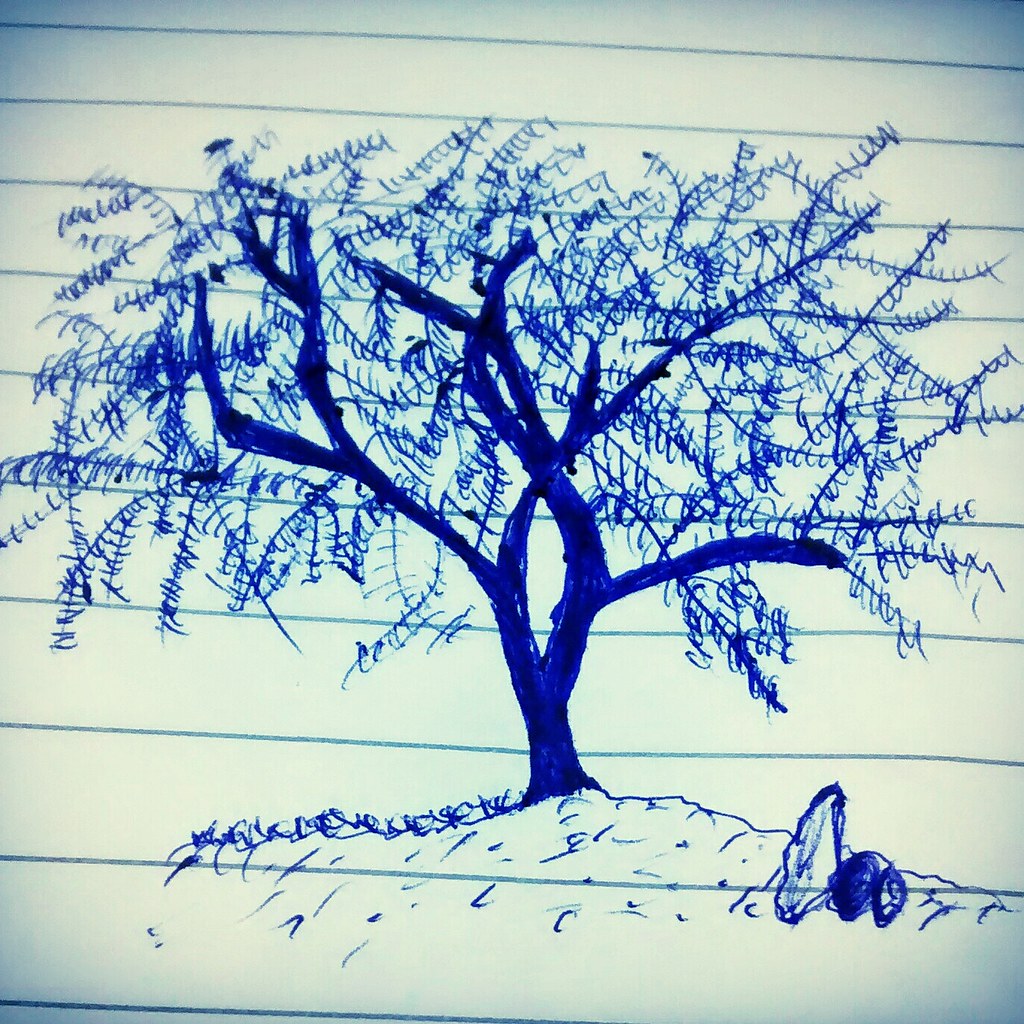On a white sheet of paper, there is an intricate drawing made with a royal blue magic marker. Horizontal lines, spaced about two inches apart, span the entire piece, creating a structured background. The scene begins with a small mound of dirt situated approximately two lines up from the bottom. This mound is detailed with several tufts of grass and stones on the right side—one large boulder accompanied by two smaller rocks. Rising from the mound is the colossal trunk of a tree, which splits into two major branches that twist and intertwine, creating a dynamic and intricate structure. These main branches further bifurcate, each subdividing repeatedly into a network of smaller branches adorned with numerous leaves. The detailed composition captures the natural complexity and organic beauty of the tree, juxtaposed against the geometric framework of the horizontal lines.